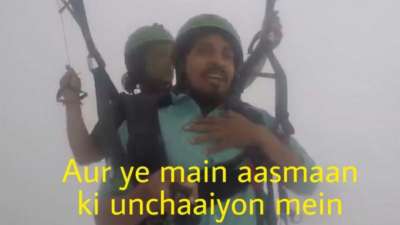The image depicts two individuals, a man and a woman, seemingly engaged in a skydiving or paragliding adventure, suspended in mid-air against a gray, cloudy background. Both are equipped with black harnesses and straps, presumably for their parachutes. The man, positioned in the front, is wearing a green hat, a turquoise polo shirt, and sports a goatee with brown skin. His left hand is placed on his chest, perhaps indicating a moment of fear or relief. Behind him, the woman is also wearing a green helmet, though her other clothing details are less visible. Yellow text in a foreign language appears at the bottom of the image, with the phrases "AUR YE MAIN AASMAA"N" and "KI UNCHAAIYON MEIN" elegantly scripted across two lines.